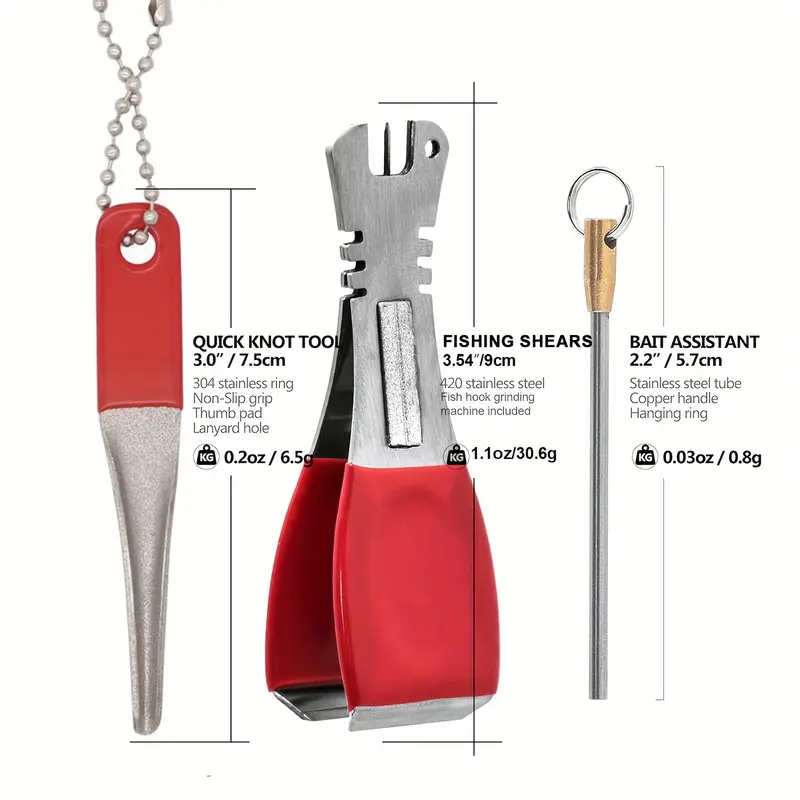The image depicts three distinct pieces of fishing equipment on a solid white background. The first tool is a Quick Knot Tool, hanging from a beaded keychain, with a red handle and a grey-silver metal section. The tool, labeled "Quick Knot Tool," measures 3 inches (7.5 centimeters) and includes features such as a 304 stainless ring, non-slip grip, thumb pad, and lanyard hole. It weighs 0.2 ounces (6.5 grams). 

Next to it is a pair of Fishing Shears with a red grip and silver metal components. It measures 3.54 inches (9 centimeters) and is made of 420 stainless steel. This tool also includes a fish hook grinding machine and weighs 1.1 ounces. 

The third tool is a Bait Assistant, characterized by its golden handle with a ring and an extended silver metal section. This slim and straightforward tool is 2.2 inches (5.7 centimeters) long and weighs 0.03 ounces. It's adorned with a copper handle that includes a hanging ring, ideal for attachment purposes.